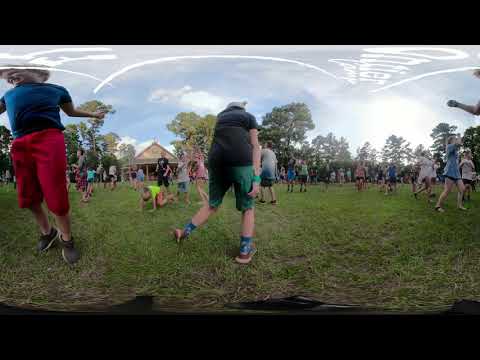This panoramic, fisheye image captures a vibrant outdoor scene at a lively festival or gathering on a partly cloudy day. The grassy field, dotted with patches of brown, stretches out beneath a bright blue sky with white and gray clouds. In the bright sunlight, children and adults alike are seen energetically running, walking, and dancing in various directions. Central to the image is a child facing away from the camera, dressed in a black T-shirt, green shorts, blue patterned socks, and red sneakers. To the far left, another boy with blonde hair, wearing a blue shirt, red shorts, and dark shoes, can be seen looking off to the side, with his arm visible on the right edge of the panoramic view. In the background, a small pavilion or gazebo stands amidst a scattering of trees, marking the distant edge of the field. The participants, adorned in a rainbow of summer clothes – reds, blues, greens, and yellows – contribute to the joyous, dynamic atmosphere captured in this immersive photograph.